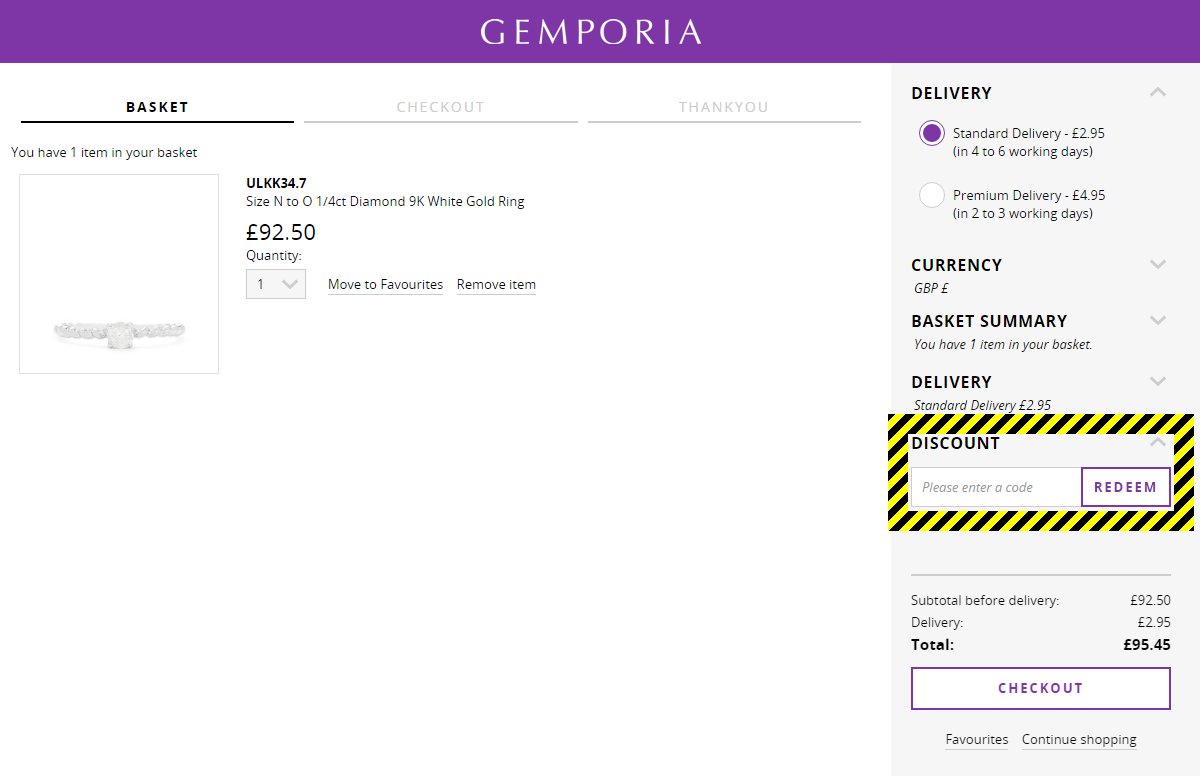Screenshot of Jimpora Website Checkout Page:

This image is a detailed screenshot of a checkout page on the Jimpora website. At the very top, there's a distinct purple border. The left section showcases the item being purchased: a 9-carat diamond white gold ring listed at £92. The ring appears silver with a prominent diamond at its center, accompanied by an image for clarity.

To the far right, delivery options are displayed, with the user choosing standard delivery over premium. Below, a notable section with black and yellow diagonal stripes stands out, indicating a discount code input area.

In the bottom right corner, the checkout details are clearly visible. The subtotal before delivery costs is £92.50, the delivery fee is £2.95, and the final total amounts to £95.45.